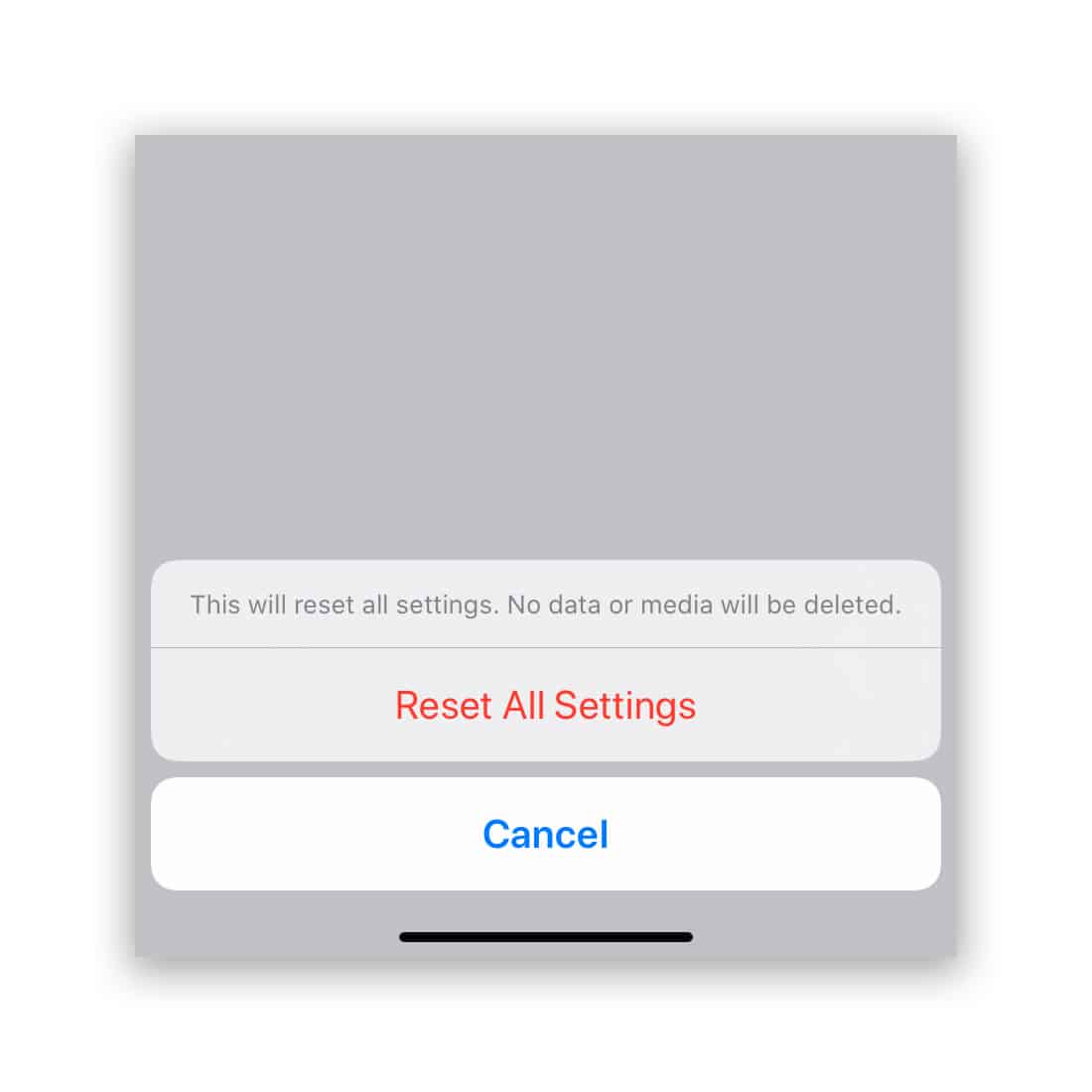The image is a screenshot with a non-detailed layout and a gray background that diffuses at the edges. The screenshot prominently features two rectangles. 

The top rectangle is a lighter gray with rounded corners, divided into two sections by a light gray line. In the upper section, a message reads, "This will reset all settings. No data or media will be deleted." Beneath this statement, in large red font, it states, "Reset All Settings."

Just below this is a white rectangle, also with rounded edges. Inside this rectangle, in bold blue font, is the word "Cancel," and directly below it, a bold black line spans the center third of the row.